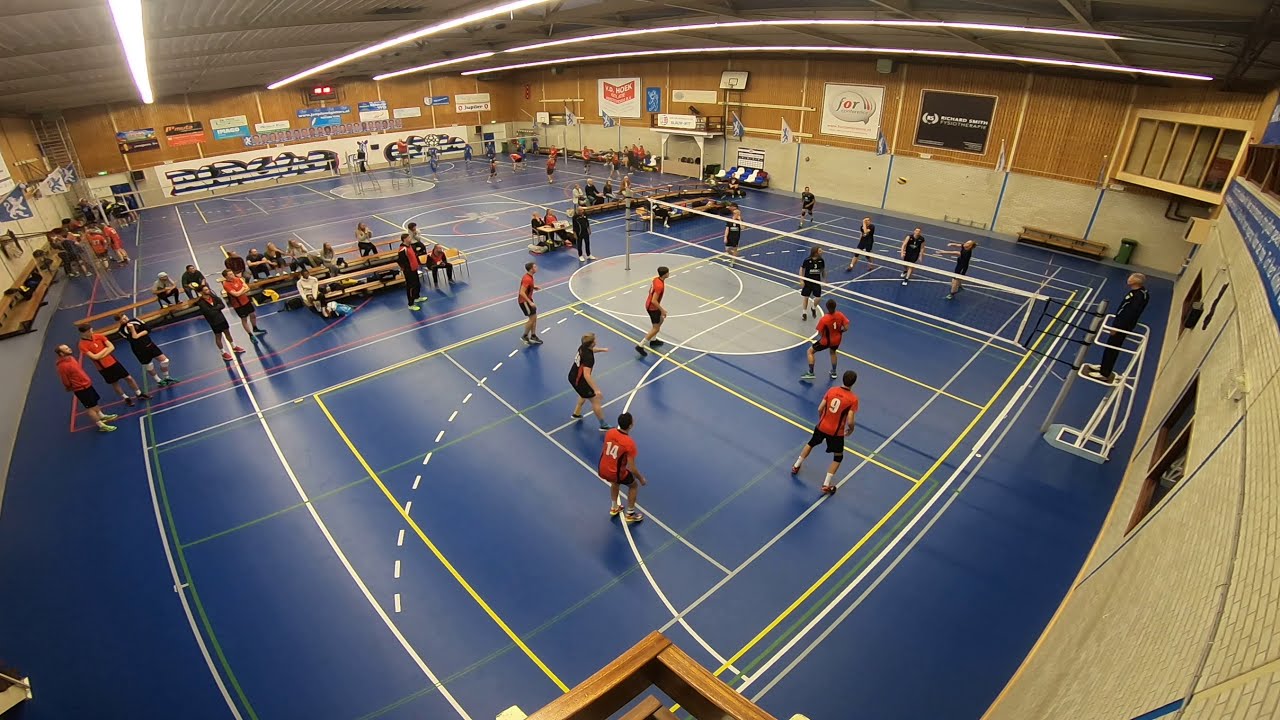The image captures a detailed aerial view of an indoor high school boys' volleyball game in a large gymnasium. The gym floor is a striking deep blue, marked with white, yellow, and green lines indicating boundaries and zones. The scene is centered around a close volleyball court angled slightly away from the viewer. On this court, a referee stands on a white platform, dressed in black, perched on gray posts, overseeing the match. 

The team closest to the viewer wears red jerseys with white numbers and black shorts, actively engaged in the game, possibly returning a serve. Opposing them, in the distance, is a team clad entirely in black. Both teams are locked in a spirited competition.

Dividing the primary court from a second in the background, which is currently not in use, is a section of brown bleachers filled with spectators and players from other teams awaiting their turn. The gym's structure features two-tone walls—the bottom half constructed of gray brick and the top half paneled in brown wood. Various colorful advertisements and banners hang from the walls, adding vibrancy to the setting.

Overall, the energy and dynamics of this volleyball game are captured with spectators intently watching, while in the far background, another match unfolds simultaneously on the second court, illustrating the bustling and competitive atmosphere of the athletic center.